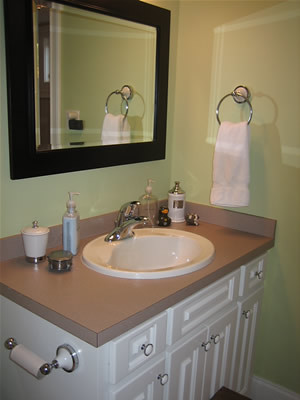This photograph showcases a small, well-organized bathroom. Central to the image is a bathroom mirror with a distinctive black frame. Below the mirror sits a white ceramic sink, complete with a sleek silver faucet and a temperature-adjusting handle. The brown countertop around the sink is scattered with various bottles and personal items. 

Beneath the countertop, there are drawers and cupboards adorned with white knobs featuring silver accents. Positioned in the lower left corner of the image is a toilet paper roll, mounted on a silver and white fixture with a metallic bar for easy replacement.

The mirror reflects a towel hanging from a towel rack, exhibiting a matching white and silver design. The greenish wall background, accompanied by a white baseboard along the floor, creates a cohesive aesthetic. The reflection also suggests the presence of a light source in the room, adding depth by casting the mirror's silhouette onto the wall.